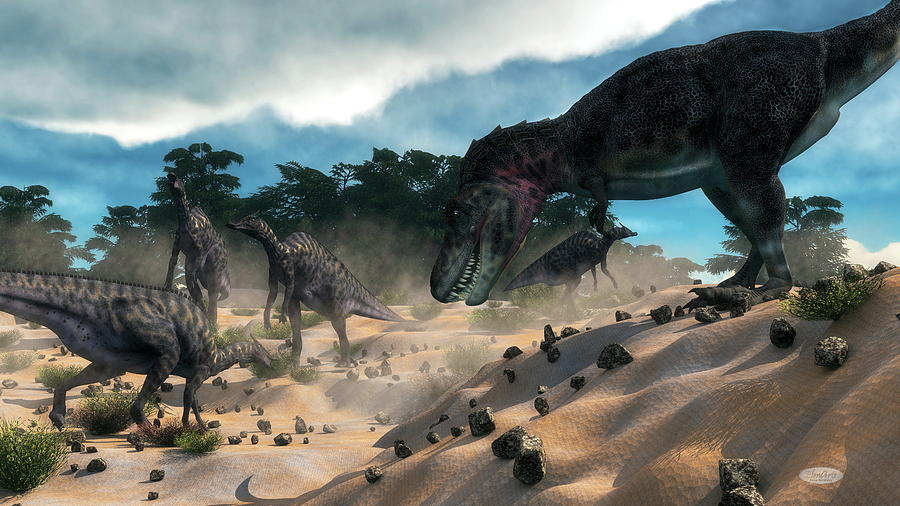A fearsome Tyrannosaurus rex dominates the scene, its sharp teeth and menacing gaze exuding raw power and aggression. In stark contrast to its imposing figure, a few smaller dinosaurs of the same species encircle the T. rex, each with smooth backs and long, slender tails. The sky above is a serene light blue, dotted with fluffy white clouds, one notably large cloud positioned in the top left corner. The ground is scattered with round stones, adding texture to the prehistoric landscape. The smaller dinosaurs, despite their size, appear wary but unified in the presence of the formidable T. rex.